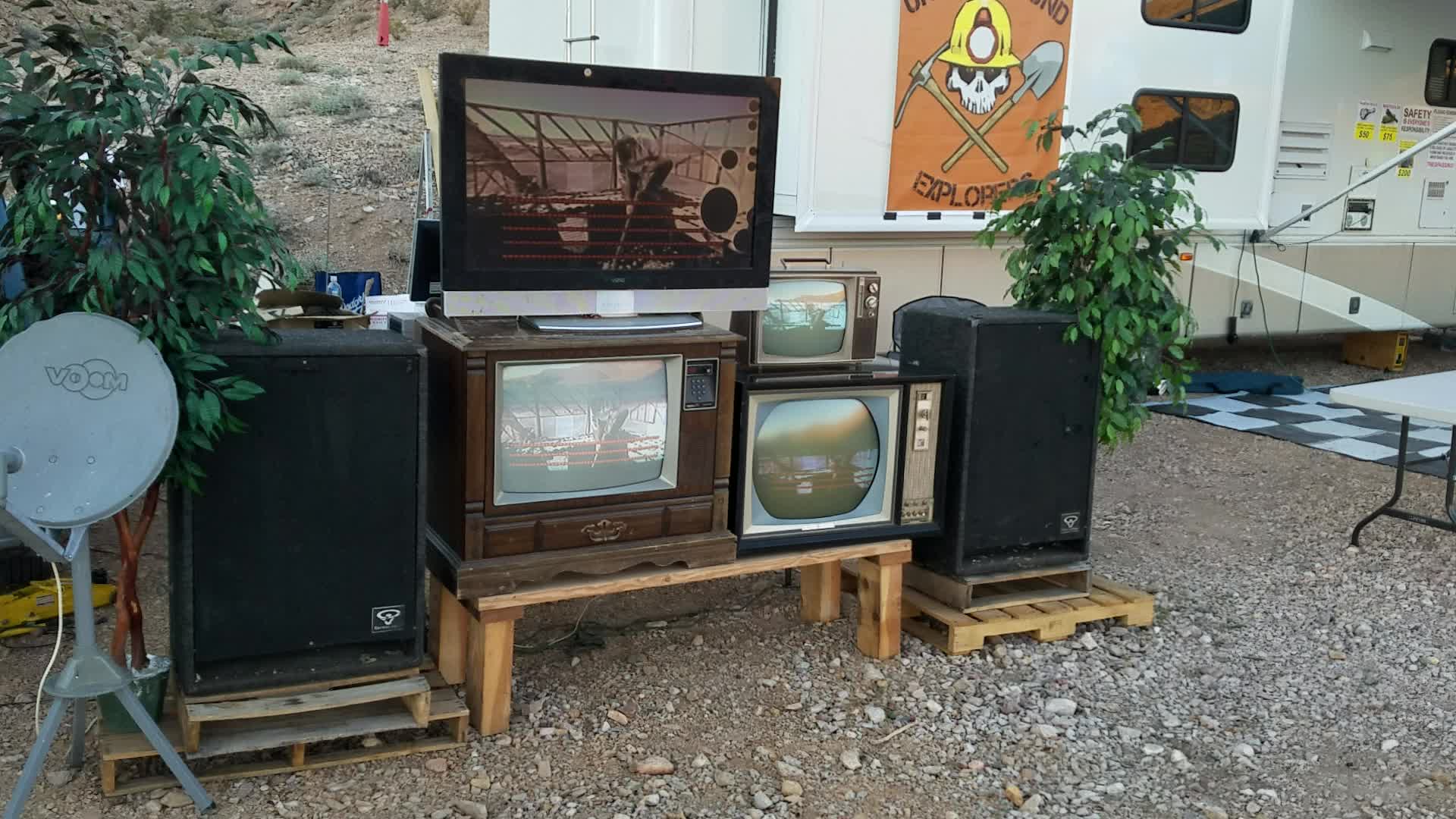The image depicts an outdoor setting with a curious mix of old and new technology arranged in front of a white wall featuring windows and a poster with a skull wearing a miner's hat, labeled "Explorers" accompanied by a pickaxe and shovel. Positioned on flat wooden crates or pallets is a collection of vintage TVs: a brown box TV, another with a circular screen, and a smaller box TV, all seemingly classic models. And above these are a more modern flat screen monitor and two large, speaker cabinets, which look like they might be used for bass guitars. A satellite dish is located to the left, flanked by two potted plants, adding a touch of greenery. Scattered wires and poles are visible on the wall, enhancing the impression that this scene is part of a movie or show set, possibly with fake or prop items. The ground is covered in gravel, and there is a hill in the background, which further cements the outdoor ambiance despite the indoor decorative elements.